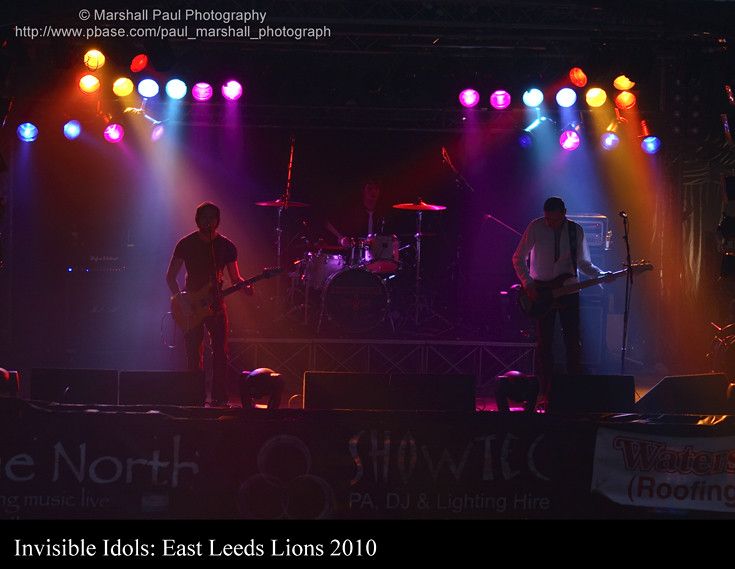The photo captures a vibrant, dynamic scene of a band performing on stage at a darkened nightclub or concert hall. Two guitarists are positioned at the front of the stage; the one on the left is a singer/guitarist dressed in a black shirt and black pants, playing a Fender guitar and singing into a microphone. The guitarist on the right is a bass player, distinguished by his black bass guitar, black pants, and white shirt, with his bass rig behind him perched on an elevated riser. A drummer, barely visible in the back middle, plays a set of silver drums with a prominent black bass drum. The stage is bathed in a kaleidoscope of colors from overhead lighting, featuring blue, purple, pink, yellow, red, and orange hues, contributing to the energetic atmosphere. At the bottom of the stage, a banner reading "North Show Tech PA DJ and Lighting Hire" is partially visible, while another banner indicates "Invisible Idols, East Leeds Lions 2010." A copyright notice at the top attributes the photo to "Marshall Paul Photography" with a website link provided.